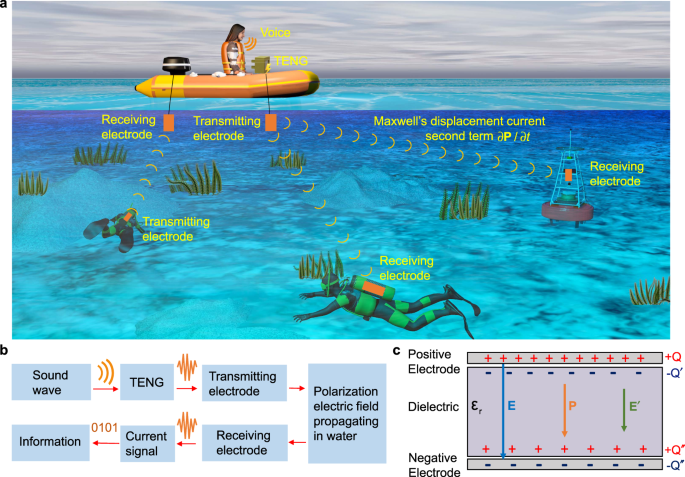This computer-generated diagram presents a detailed representation of sound wave transmission and communication in an underwater environment, primarily showcasing the movement and interaction of electrods. The scene includes a female figure with long hair sitting in an inflatable raft equipped with a motor. She is using a device labeled "TENG," signaled with a lightning bolt symbol, to transmit voice commands, depicted by arches emanating from her mouth, designated as "voice". The device links to a system with transmitting and receiving electrodes.

Beneath the water, indicated with grayish-blue hues, several scuba divers are situated. These divers are equipped with tanks featuring orange-colored devices marked as either transmitting or receiving electrodes. The diagram traces the path of the sound waves as information travels from the raft's device, through the water via the electrodes, ensuring communication between the person in the raft and the divers below.

Additional annotations include technical terms such as "Maxwell's displacement current, second term," highlighting the scientific aspect of the diagram. Arrows and orange lines visualizing the data flow, further illustrating how the polarization electric field propagates in water, effectively transmitting the current signal and information. Labels at the bottom reiterate this process, incorporating details like "positive electrode," "dielectric," and "negative electrode." The detailed presentation emphasizes the cycle of transmitting electrods and how vital underwater communication relies on this systematic propagation of sound waves and electronic signals.